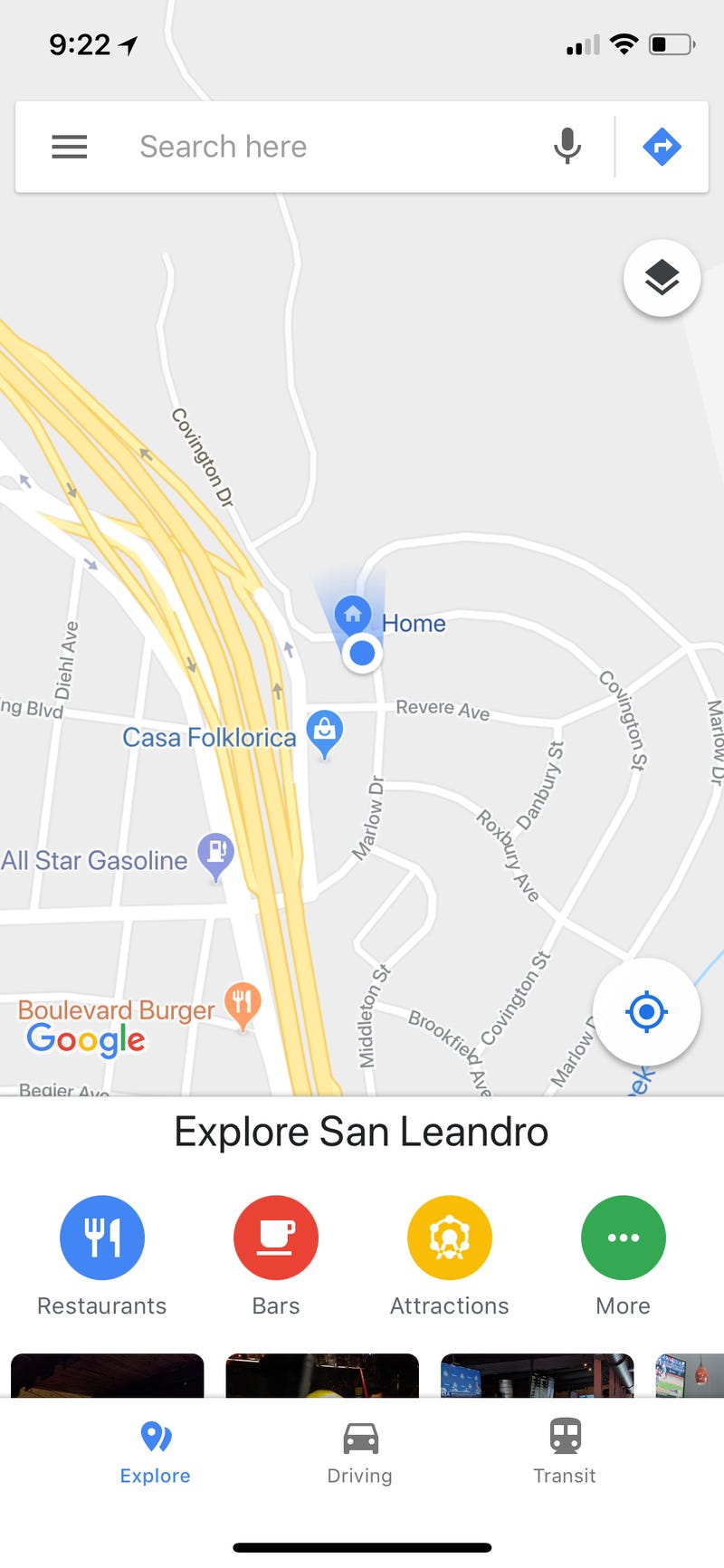This image is a screenshot of the Google Maps app displayed on a mobile phone in portrait orientation. The mobile phone's interface shows the time as 9:22 in the upper left corner, with the signal strength indicated by two bars and the battery level at approximately one-third capacity in the upper right corner. Below these indicators, there is a white search bar positioned against a gray background.

The map itself is characterized by white roads, yellow highways or freeways, and dark gray text labeling various street names. Several pins mark key locations on the map, including a gas station, a restaurant, a shopping destination, and a blue pin representing the user's home. The user's current location is indicated by a dot precisely over the home pin.

Directly beneath the map, the text "Explore San Leandro" is displayed. Below this text are four rounded, colorful buttons: blue for restaurants, red for bars, yellow for attractions, and green for more options. The very bottom of the screen features cut-off photograph thumbnails, hinting at additional visual content. Finally, there are navigation tabs situated at the bottom of the screen, offering options to switch between explore, driving, and transit modes.